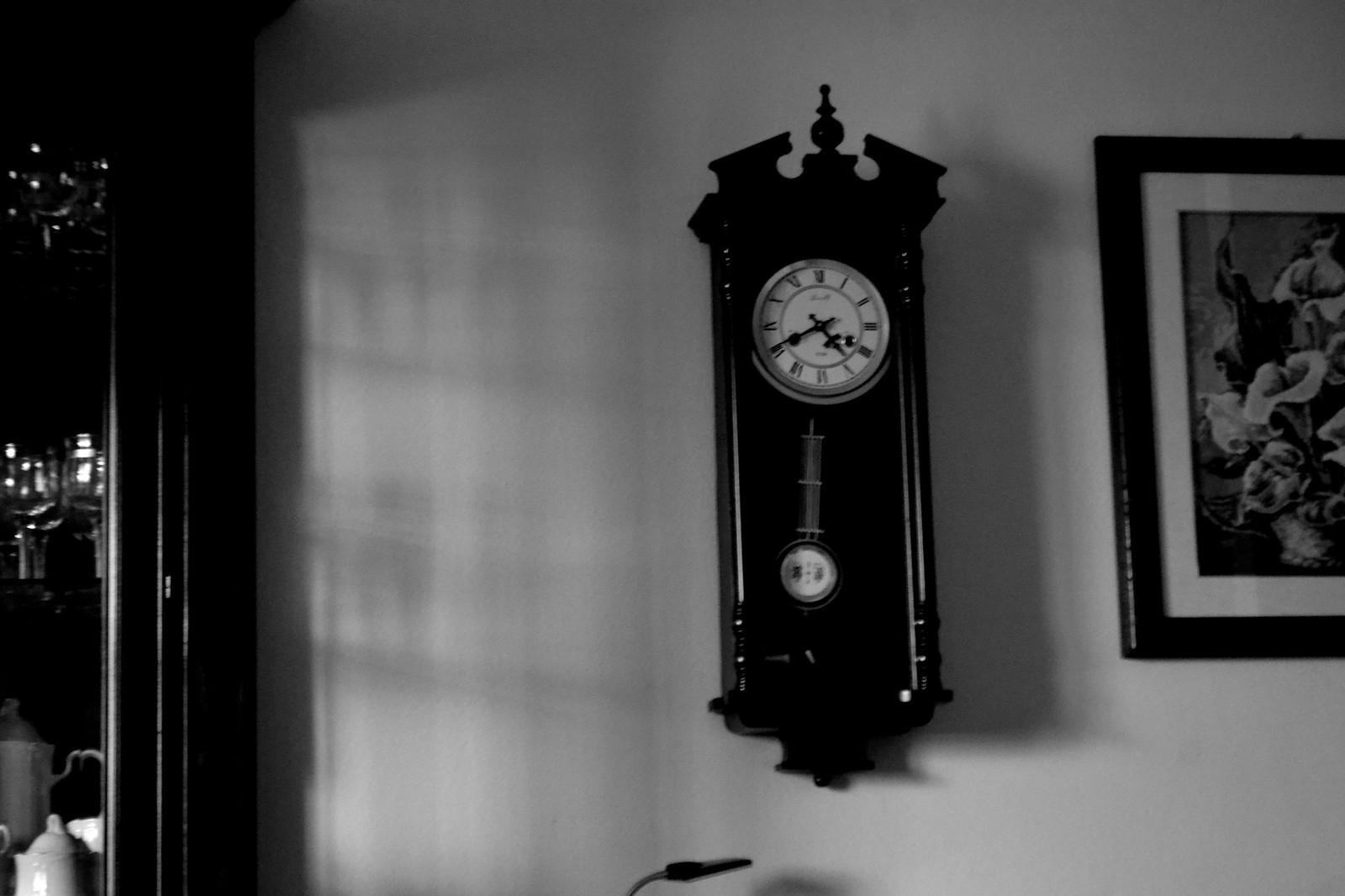The black and white image captures a traditional miniature grandfather clock mounted on a white wall. The clock, appearing to be made of wood but rendered in grayscale, features a prominent black case and a white clock face adorned with Roman numerals and black hands. Beneath the clock face, a short pendulum is visible through a clear glass window, with a white circular ornament featuring intricate gray artistry or writing at the bottom. To the right of the clock hangs a framed floral print, showcasing tulips, enclosed in a black frame with a white mat. On the left side of the image, a china cabinet is visible, containing three shelves. The top two shelves display silver pieces, while the third shelf houses a large teapot, a miniature teapot, and some white china or porcelain cups alongside a potential glass ornament. At the very bottom of the image, part of a black lamp with a curved neck is slightly visible. The clock reads approximately 4:40, possibly in the afternoon, though the grayscale renders the time of day ambiguous.